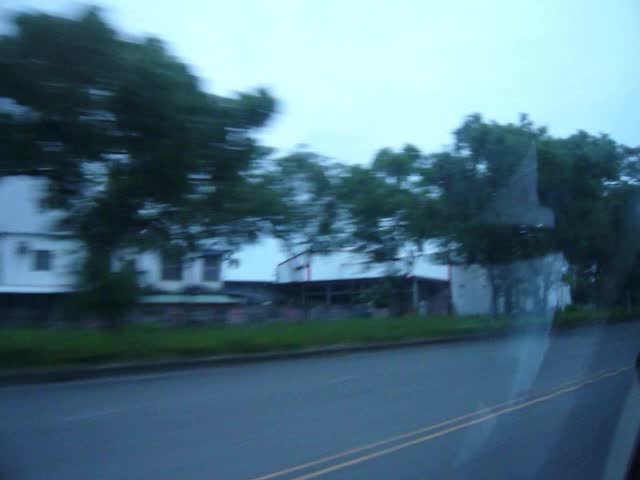This image, taken through a large window of a moving vehicle—likely a bus—depicts a slightly blurry scene during dusk. The window glass, identifiable by a faint reflection in the bottom right, reveals a two-lane road marked by two yellow median lines to the right side of the frame. Adjacent to the road, there is a lush grassy strip leading up to a series of white buildings. 

On the far left, a prominent white house, distinguished by its farmhouse-style windows and a porch with a roof, stands partially obscured by a large oak tree. Adjacent buildings also appear white, with one resembling a barn or warehouse featuring a brown, covered shed area supported by posts. These structures seem more industrial or business-oriented rather than residential. The image, with its slightly darkened ambiance, suggests that it might have been taken at the onset of evening.